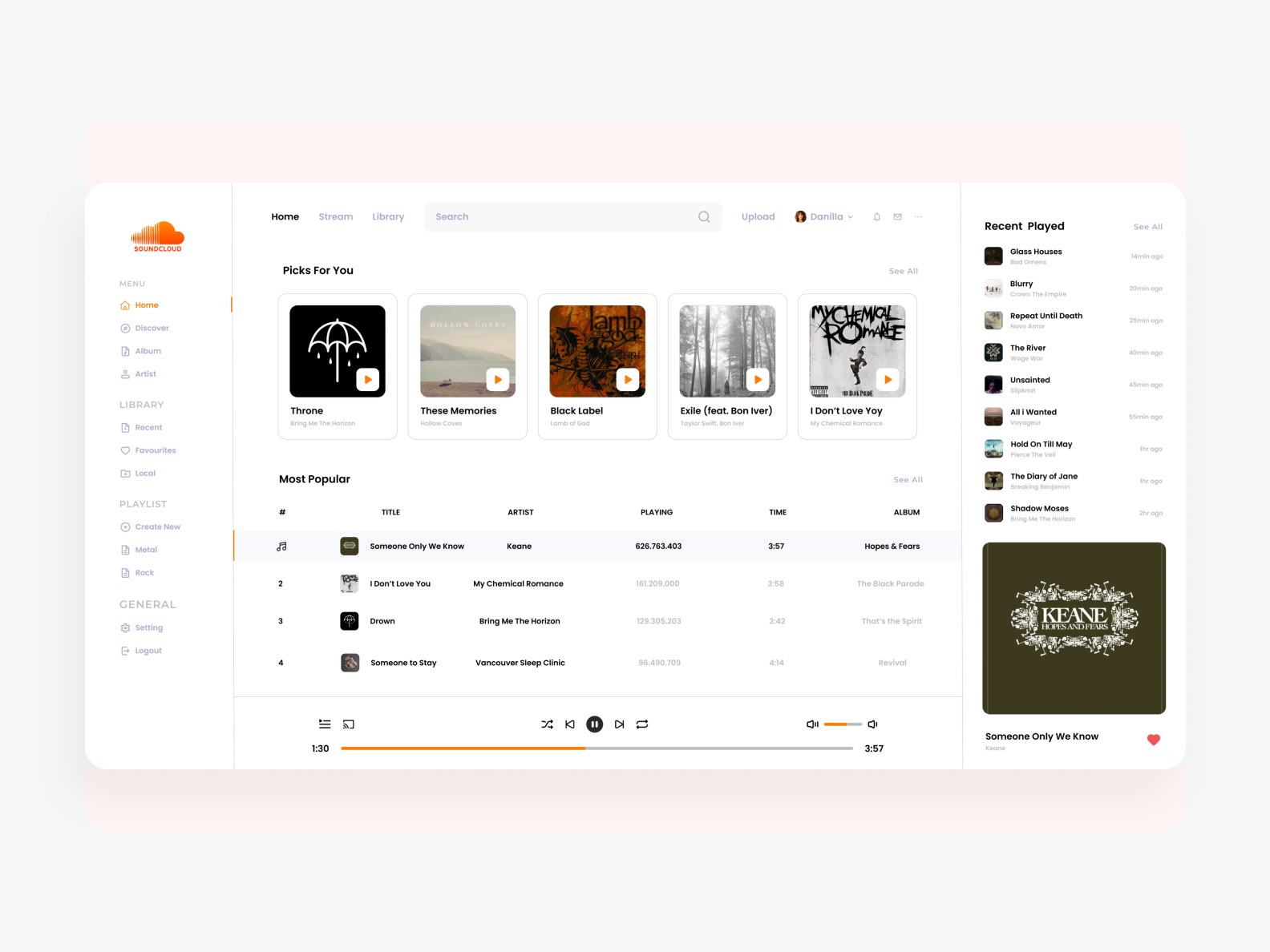The image displays the SoundCloud app interface with a very light pink background. Central to the design is a white square with softly rounded edges, indicating the main application area. The user, "D-A-N-I-E-L-A," is logged in.

In the top left corner, the SoundCloud logo is prominently displayed. Adjacent to it on the left side is a navigation bar menu that provides access to various sections such as Albums, Artists, Library, Playlists, and General Settings. The bottom of this menu houses the logout button.

The central portion of the interface highlights music recommendations, featuring various suggested albums. Although the album titles are somewhat hard to read, one standout recommendation is "I Don't Love You" by My Chemical Romance. This section presents the album art in a series of five square thumbnails. Below this section lies the play bar, offering controls for audio playback including pausing, skipping songs, replay, shuffling, and volume adjustments.

To the right side of the screen, the app displays a list of recently played songs. At the very bottom right, there is a notably larger album art thumbnail, signifying the most recently played song.